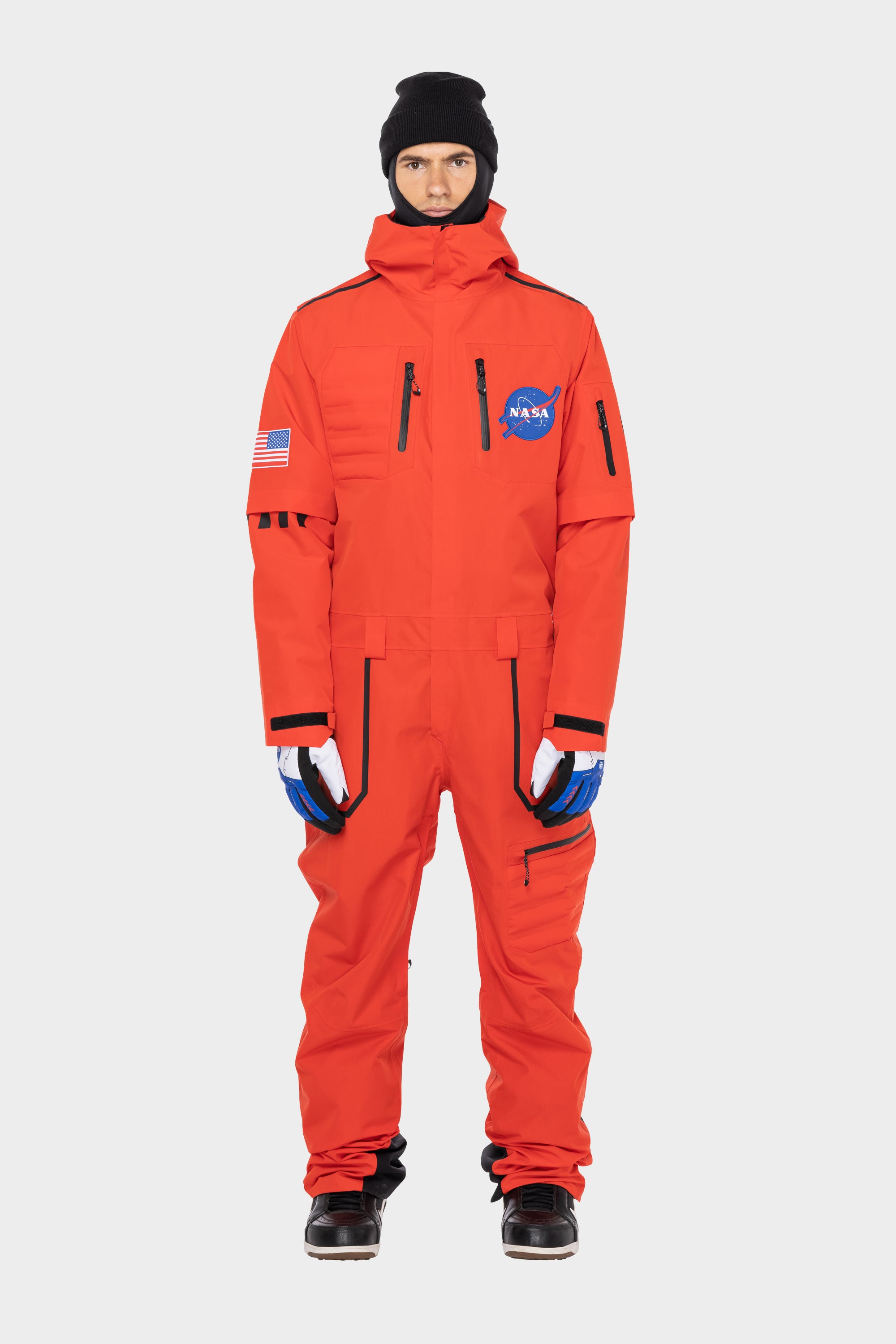This photograph features a man standing against a completely blank, white background with a subtle grey tone. He is facing the viewer directly, wearing a bright orange jumpsuit with a high collar that encapsulates his entire neck and extends down to his feet. The jumpsuit is adorned with an American flag patch on his left shoulder and a blue NASA logo patch with white lettering on the right chest area. The suit appears somewhat loose-fitting and is equipped with numerous zippers, including on the chest, left arm, both thighs, and especially notable one running horizontally across the left thigh.

The man is also wearing a black head covering that resembles a ski cap, leaving only the top of his face visible from just above the eyebrows to below the bottom lip, revealing a slightly grumpy or frowning expression. His hands are protected by gloves colored in shades of white, blue, and a touch of black. His shoes are primarily black with a bit of white detailing at the bottom.